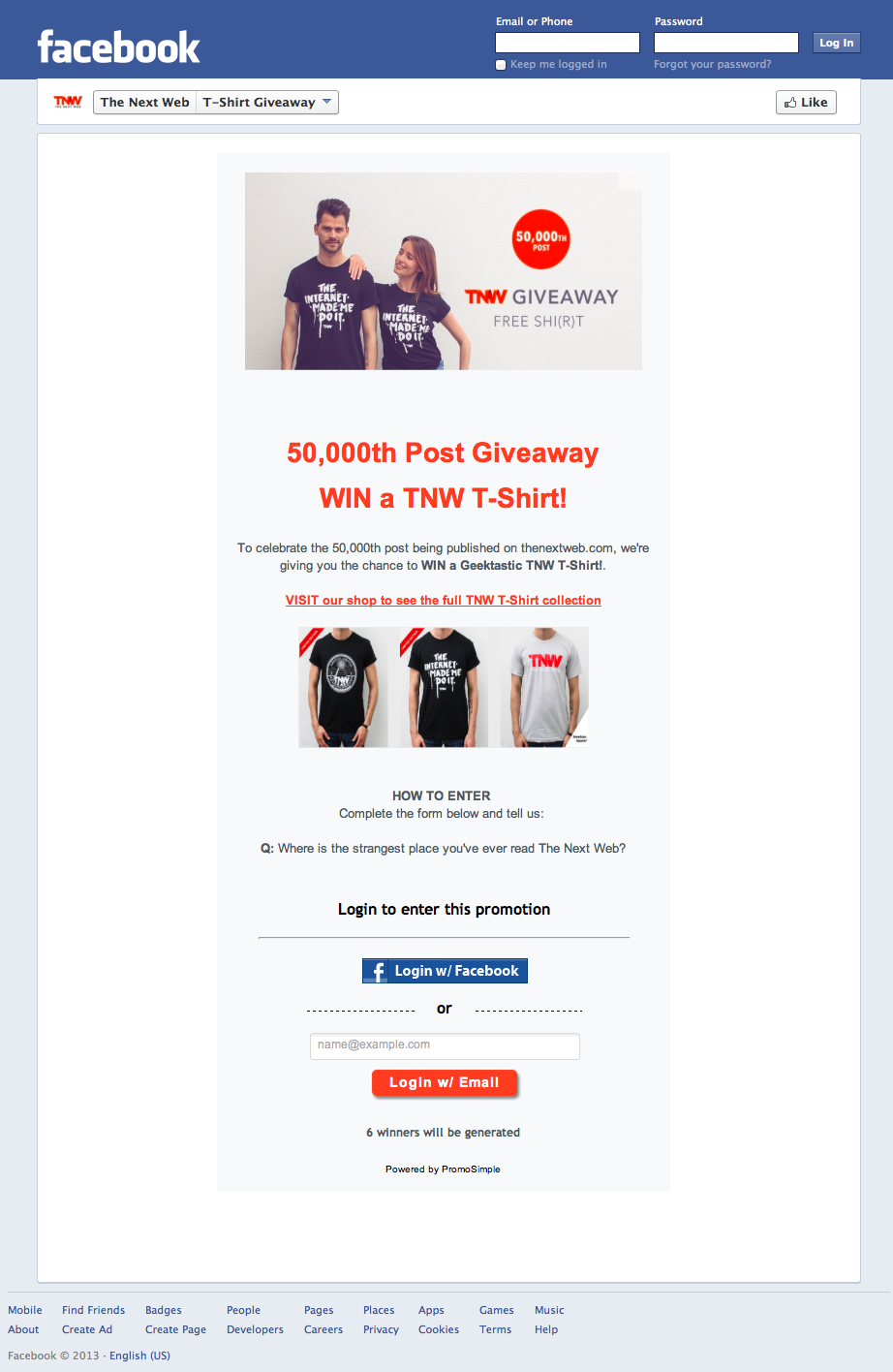The image depicts the Facebook page for TNW (The Next Web), prominently featuring a t-shirt giveaway promotion. The interface allows users to log in and interact with the page. Central to the promotion is the opportunity to win a TNW t-shirt, available in black with various designs or a white version featuring the TNW logo. Participants are encouraged to enter a contest by answering the question, "Where's the strangest place you've ever read The Next Web?" The giveaway aims to generate engagement, promising that six winners will be selected. The page also provides a form with instructions for entry and further details about the promotion, which appears to be powered by a third-party promotional service.